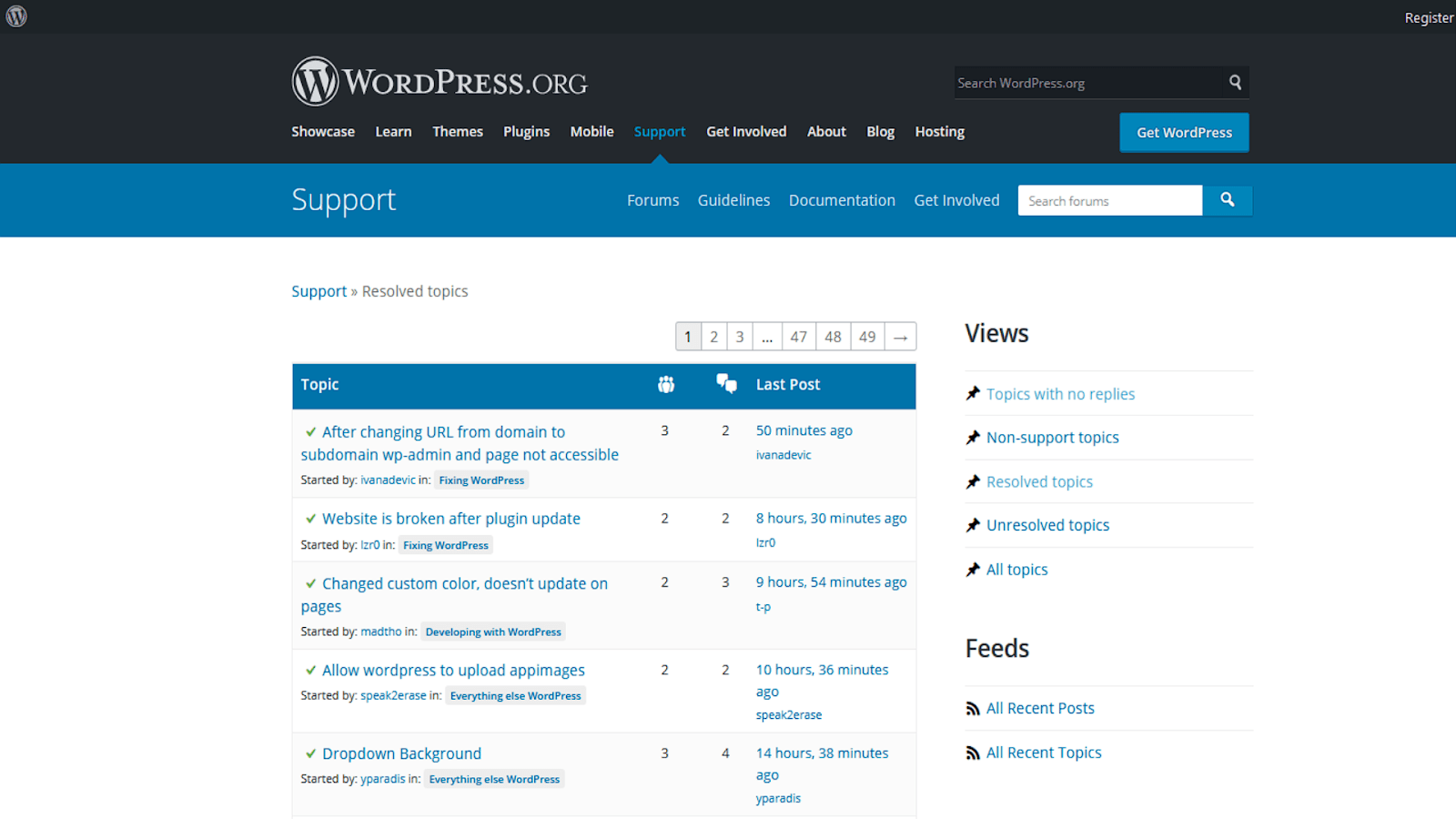The image displays the WordPress.org logo, which consists of a stylized white "W" inside a white circle, all set against a black background. Below the logo, the words "WordPress.org" are prominently featured. Encased within the black background are various sections labeled: "Showcase," "Learn," "Themes," "Plugins," "Mobile," "Support," "Get Involved," "About," "Blog," and "Hosting."

Adjacent to this section, there is a teal-colored button labeled "Get WordPress." Beneath this primary button is another teal box labeled "Support," which presents additional options: "Forums," "Guidelines," "Documentation," and "Get Involved." An empty search bar labeled "Search Forums" is located nearby, with an arrow pointing towards the "Support" section.

Below these navigational elements, the forum topics are highlighted in a teal-colored bar, listing the "Topic" and "Last Post" times. The following forum titles and corresponding timestamps are included:
1. "After changing URL from domain to subdomain, wp-admin, and page is not accessible" – posted 50 minutes ago.
2. "Website is broken after plugin update" – posted 8 hours and 30 minutes ago.
3. "Change custom color doesn't update on pages" – posted 9 hours and 54 minutes ago.
4. "Allow WordPress to upload app images" – posted 10 hours and 36 minutes ago.
5. "Drop-down background" – posted 14 hours and 38 minutes ago.

The image comprehensively outlines the primary navigation and recent forum activity available on WordPress.org, highlighting common user concerns and support options.